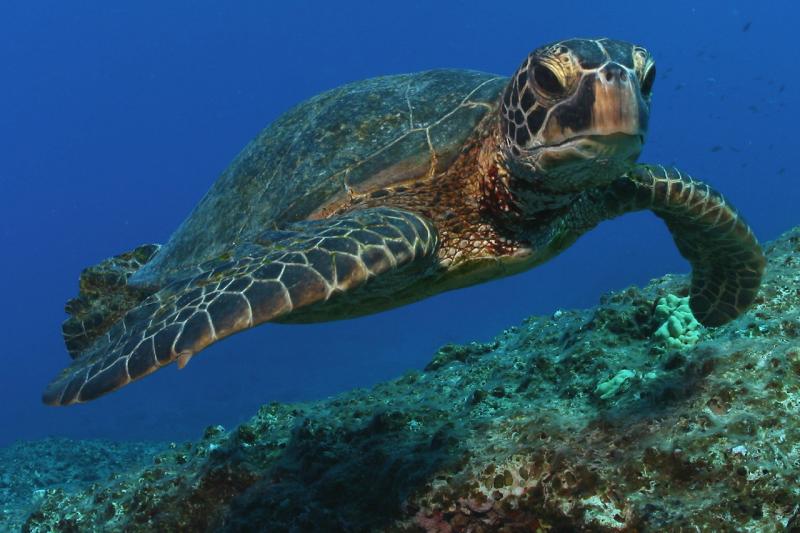This vibrant image captures a large sea turtle swimming gracefully in the deep, beautiful blue water. The turtle's head, adorned with dark eyes surrounded by brown patches, and a greenish-tint on the top, is looking towards us with its nose pointed forward. Its flippers, slightly curved backward, exhibit a dark green color with intricate white lines running down their length, similar to the patterns on its shell, which is a striking shade of green marked with white lines. Beneath the turtle, a porous seabed covered with green algae and some brown patches of coral or rock is plainly visible. The background is dominated by the deep, dark blue of the ocean, enhancing the overall serenity and beauty of the scene.